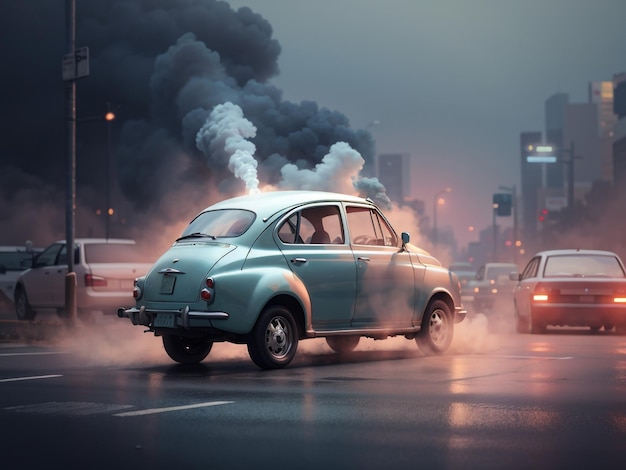In this digital rendering, a light blue car akin to a Mini Cooper, but with a rounded Volkswagen-like shape, sits prominently on a wet road, facing right. Emitting from the car's roof are white films that ascend into the air as dense black smoke, particularly concentrated in the top left corner. The scene, set at evening, features a dark, grayish-blue sky. Surrounding the central car, multiple vehicles travel the road, their headlights casting reflections on the wet pavement. To the extreme left, there's a glimpse of a parking lot. In the distant background, a series of tall buildings are visible under the artificial streetlights, highlighting an atmosphere of an ongoing disaster with billowing smoke suggesting a large fire. The color palette is dominated by aqua, gray-blues, whites, grays, blacks, and hints of orange from the streetlights.